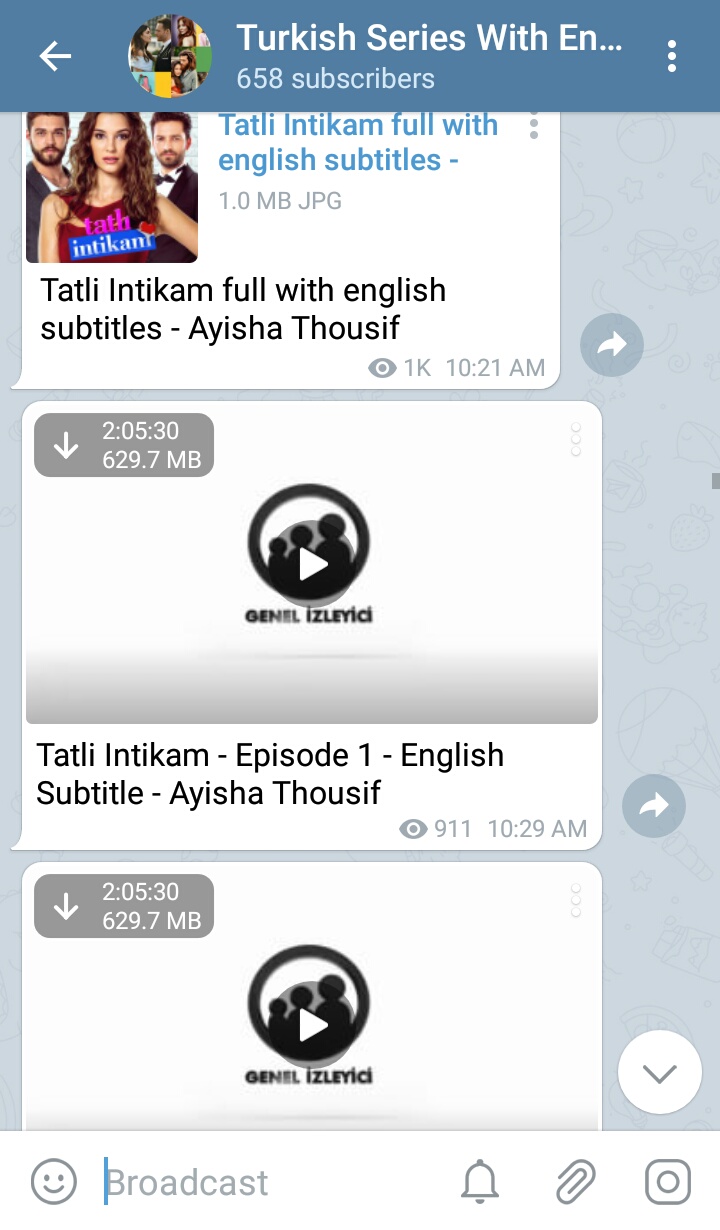This image appears to be a screenshot from an application, featuring content related to a Turkish series. At the top of the screen is a blue header bar. On the left side of this bar is a white arrow pointing to the left. Next to the arrow, there is a circular thumbnail photograph, which appears to contain multiple people, but the details are not clearly visible. The text on this blue bar, in white font, reads "Turkish series with EN...". To the right, it shows that the series has 658 subscribers, and there are three vertically aligned bold dots in the top right corner, presumably a menu icon.

Below the blue bar, there is an image occupying a considerable portion of the screen. This image showcases a woman flanked by two men, one on each side, standing just behind her shoulders. The woman has chestnut-colored, wavy hair that falls past her shoulders. Both men have mustaches and beards, giving them a distinguished look.

Underneath this photograph, there is a descriptive text inside a white speech bubble. The text, in black font on a white background, says "Tatli Intikam, full with English subtitles - Ayesha, Thusif." Another speech bubble is present below this one, which contains an icon with a play button, indicating media content ready to be played.